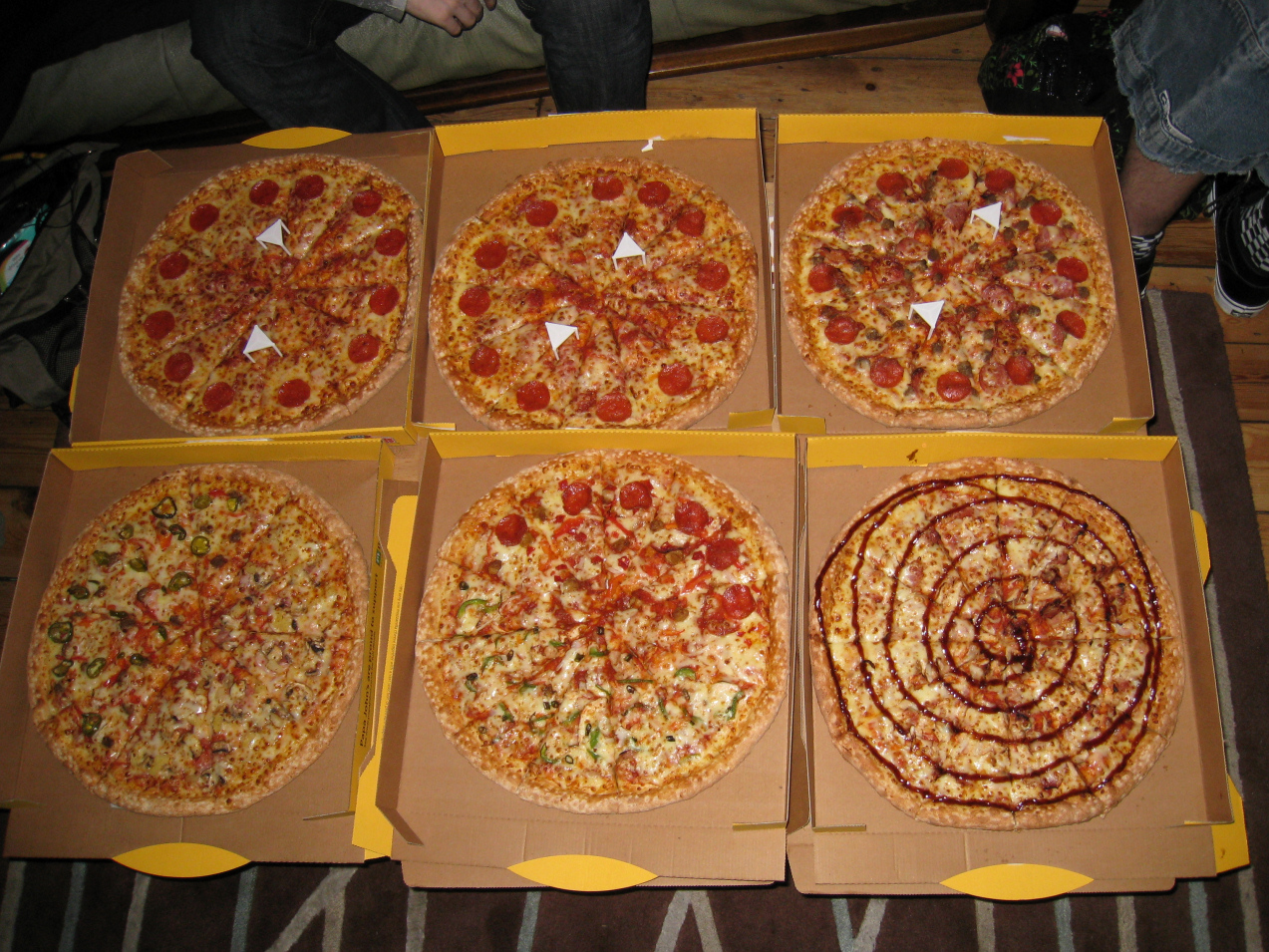This is an overhead photograph showcasing six large pizzas in their boxes, arranged in a 3x2 grid on a surface that appears to be a coffee table, partially visible against a dark brown rug with white streaks. The six pizzas feature a variety of toppings and are housed in half-open boxes with yellow tops and plain cardboard interiors. At the top row, from left to right, there are two pepperoni pizzas, each supported by two little white stands, and a pepperoni and sausage pizza with stands as well. The bottom row includes, from left to right, a cheese and jalapeno pizza, a half pepperoni-sausage and half green peppers-olives combination pizza, and a barbecue chicken pizza with a distinctive barbecue swirl. Lids of the boxes are folded underneath, exposing only the bottom of the boxes. Surrounding the table, two individuals are partially visible: one seated on a couch at the top left, wearing dark jeans, and another at the top right wearing jeans or cargo shorts paired with black Vans, facing away from the viewer.